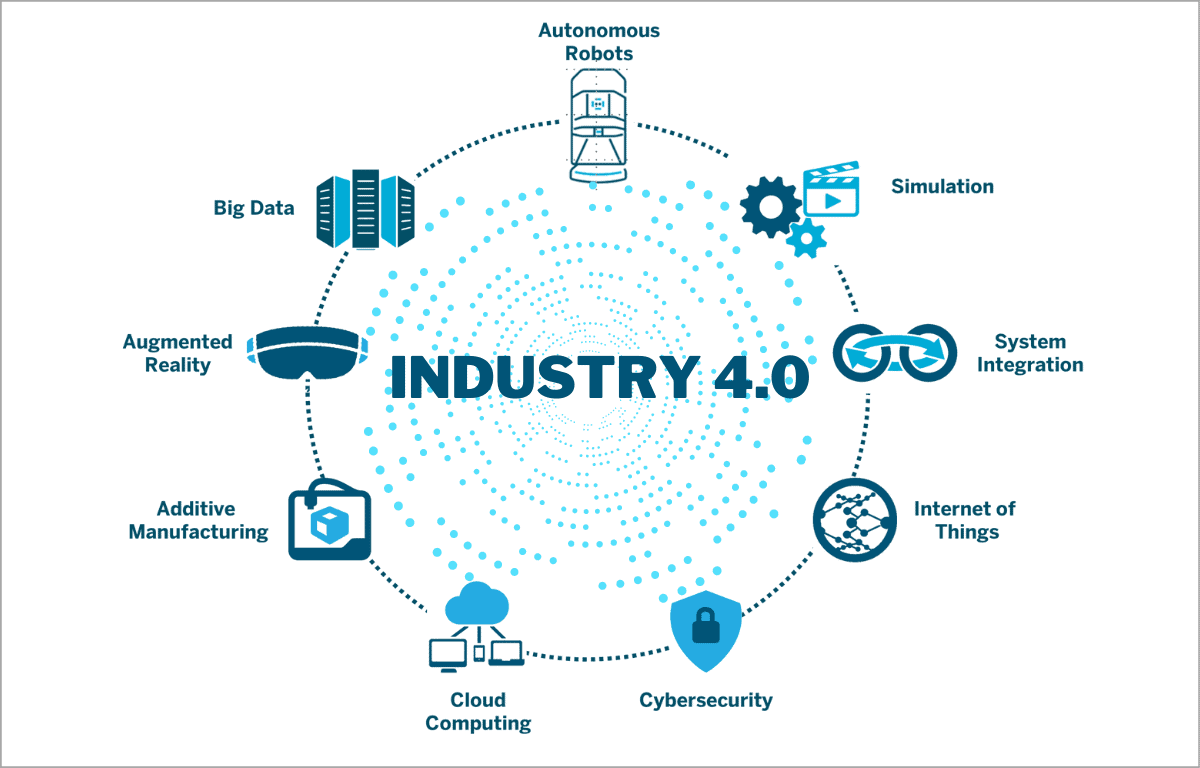The image is a detailed diagram titled "Industry 4.0," prominently displayed in dark blue letters at the center of a predominantly white background. Surrounding the central text are multiple, smaller circular icons arranged in a larger circle connected by a darker blue dot, emphasizing their interconnected nature. Beginning at the top of this circle and moving clockwise, the icons represent key components of Industry 4.0: Autonomous Robots, Simulation, System Integration, Internet of Things, Cybersecurity, Cloud Computing, Additive Manufacturing, Augmented Reality, and Big Data. Each component is accompanied by a specific icon, such as a movie reel, glasses, and skyscrapers, all linked cohesively with a consistent dark blue color scheme. The background features a subtle pattern of circular dots, adding depth to the otherwise plain white space.